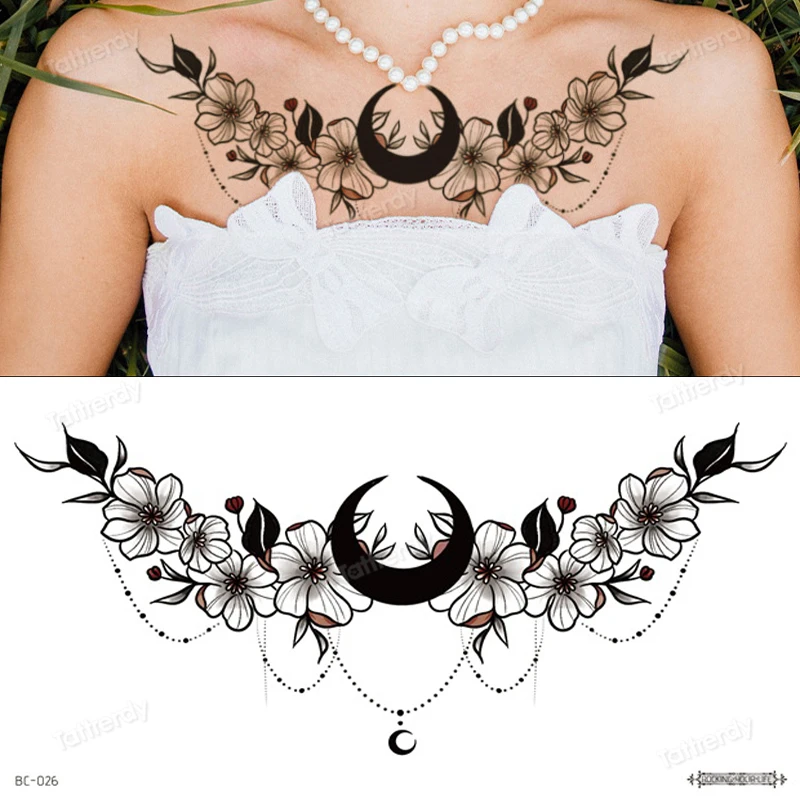The image features an intricate tattoo design on a woman's chest. The tattoo comprises a string of interconnected flowers spanning her upper chest, centered around an upside-down black crescent moon. Below the floral string, several drooping necklace-like lines arc gracefully downward, culminating in the center with a larger, dark black crescent pendant. The entire design is presented in black and white with subtle touches of red. The image is divided into two sections: the top half showcases the tattoo as it appears on the woman's chest, complete with her white beaded necklace and white dress, while the bottom half illustrates a detailed drawing of the same tattoo. The tattoo's design includes flower pedestals extending outward, linked together with chain-like connectors, and prominently features the crescent shapes at both the central and lower points of the design.